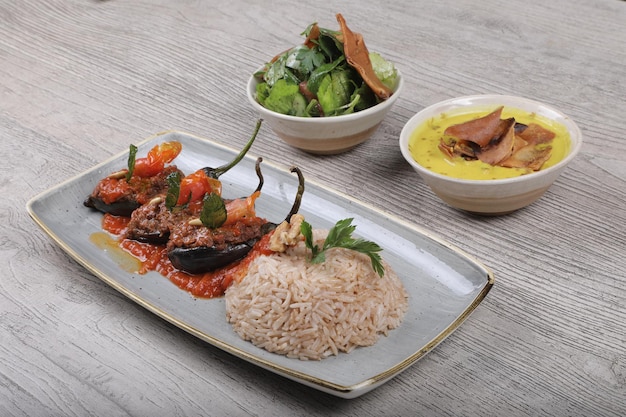On a light gray wooden table with natural dark gray lines, the image showcases three distinct dishes arranged artistically. In the bottom left, a large, rectangular silver plate holds half aubergines topped with a red, tomato-based stew, adjacent to a round mound of pilau rice, adorned with a green leaf. Above this dish, in the top center, a white bowl with a beige bottom contains a mixed green salad featuring dark green and beige elements, possibly lettuce and meat slices. To the right, another similar bowl holds a thick, yellowish soup, possibly cream-based, with folded brown pieces that could be thin slices of meat or vegetables. The overall presentation is set against the table's distinctive grainy texture.